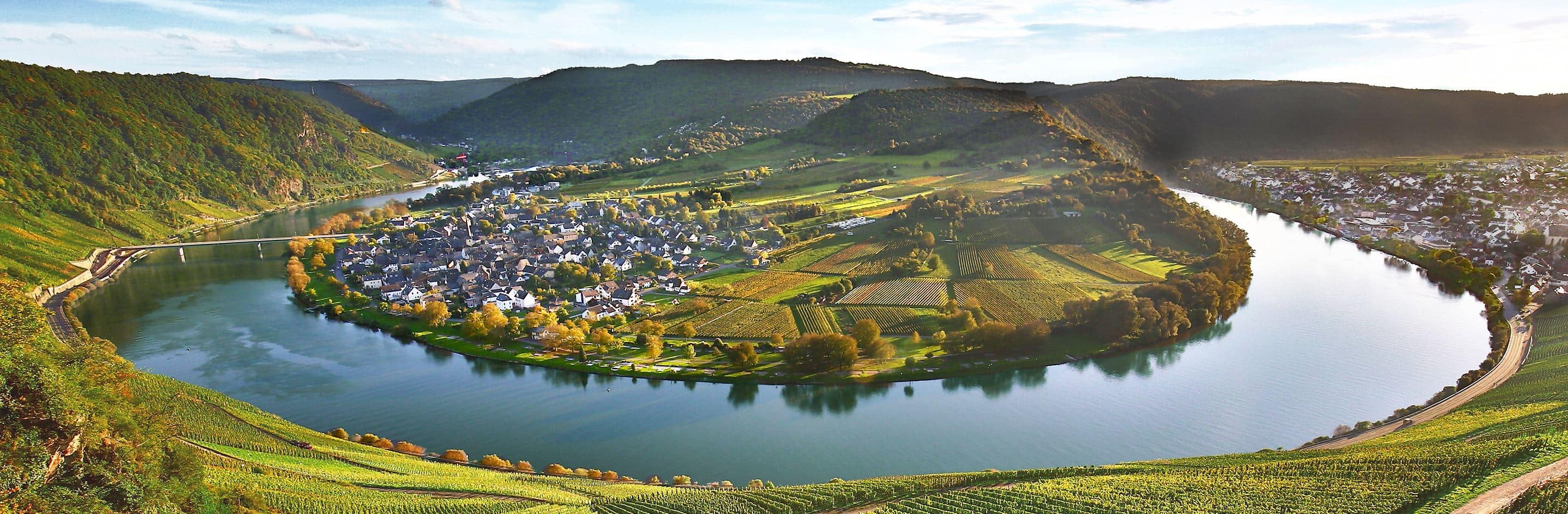This panoramic, horizontally aligned rectangular image presents a stunning aerial view of a valley town nestled within an elevated hilly landscape. The wide and relatively short picture captures a large, circular piece of land surrounded by a calm, grayish-blue river, which forms a near-perfect loop around the central island. In the backdrop, a serene sky, decorated with feathery white clouds, hovers above a range of gentle hills.

The island at the center showcases a mix of densely populated urban and open rural areas. On the left side of this landmass, close to the water's edge and near a prominent white bridge that crosses the river, a cluster of compact, white buildings forms the heart of a small community. This area gradually slopes upwards towards a slight incline dotted with additional structures.

In contrast, the right side of the island features expansive green fields, some of which appear to be vineyards or simple meadows, giving way to a more rural character. The entire scene is framed by the distant mountain ranges, creating a harmonious blend of natural and constructed elements in this tranquil and picturesque setting.